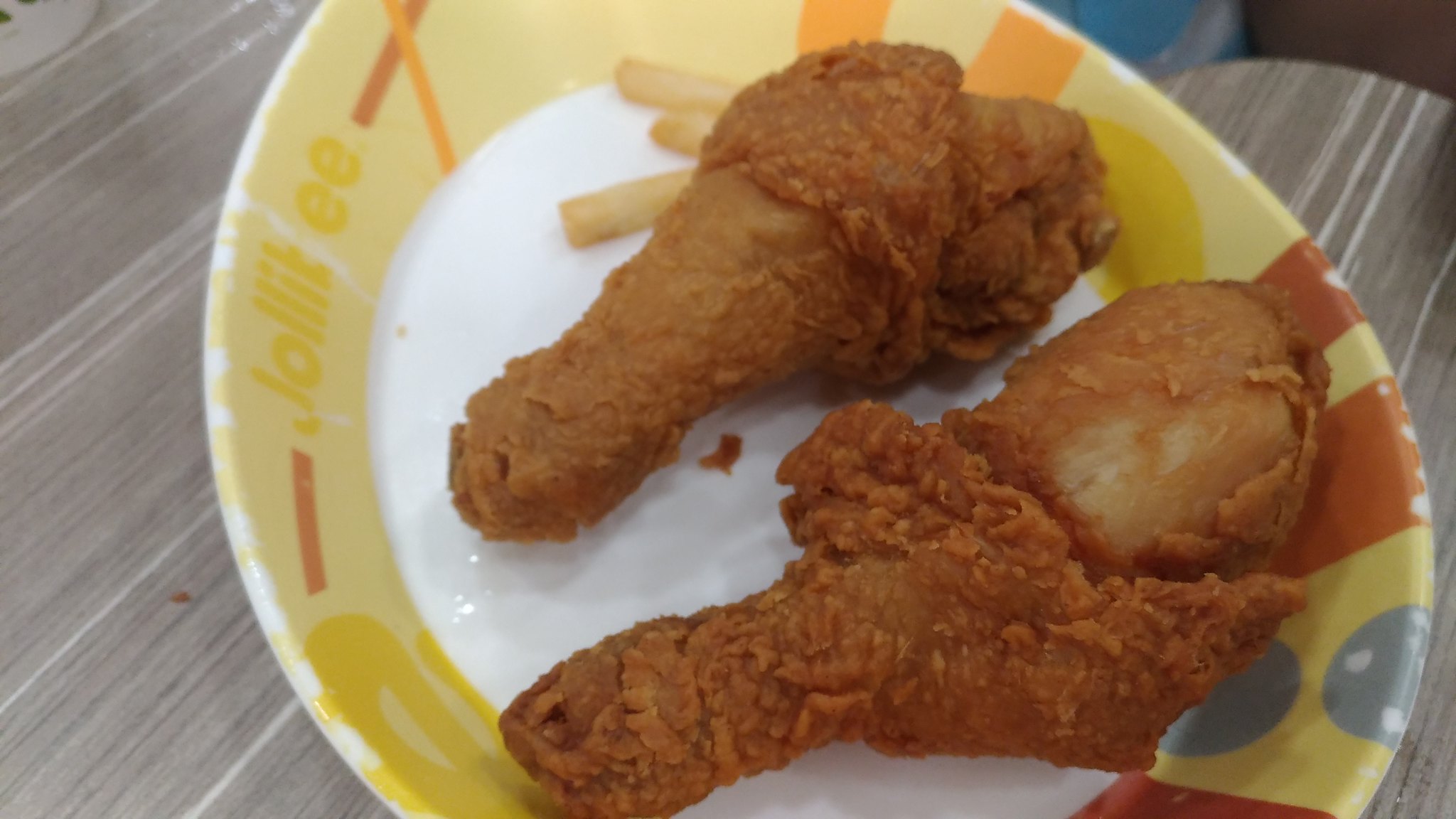This color photograph depicts a white plate with a yellow border and red stripes, inscribed with the word "Jollibee." The plate is placed on a brown wooden surface characterized by white streaks. The center of the plate features two full, crispy fried chicken drumsticks alongside a few french fries, precisely three. The drumsticks remain uneaten and appear brown and crispy, though they have cooled down and seem a bit dry. The scene suggests a budget-friendly dining experience at a casual eatery. The overall presentation, including the plain gray table surface, adds to the impression of an inexpensive meal setting.